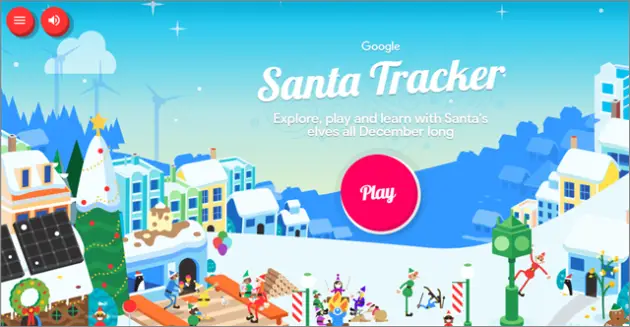Illustration Caption: 

"An enchanting winter scene unfolds beneath a serene gradient sky, transitioning from deep blue at the top to a lighter hue near the horizon, scattered with twinkling stars and gentle clouds. In the distance, wind turbines stand silhouetted against the skyline. A tranquil hillside dotted with charming houses is adorned with festive decorations. A vibrant Christmas tree, crowned with a shining star and adorned with red ornaments, stands proudly amid the snow-covered ground. Lampposts wrapped in candy cane striped decorations punctuate the scene, accompanied by Christmas wreaths adorning the sides of buildings. Jubilant figures dressed in green and red elf costumes bring life to the scene. The magical setting is highlighted by a bold pinkish-red circle in the foreground, inviting viewers to 'Play,' with the phrase 'Santa Tracker by Google. Explore, play, and learn with Santa's elves all December long' prominently displayed. A volume icon is subtly positioned in the upper left corner, completing the festive atmosphere."